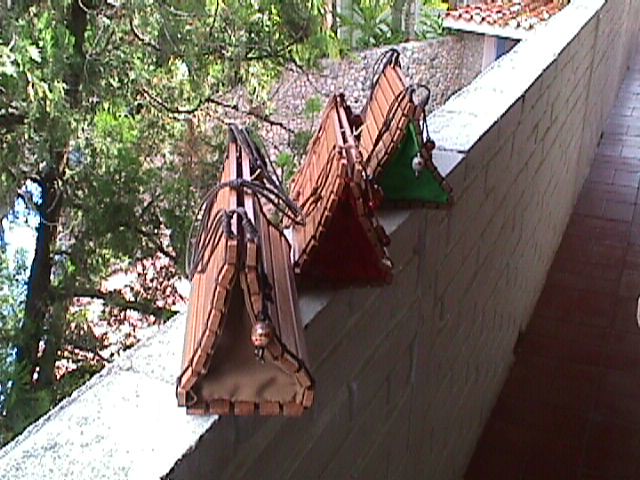The photograph captures a high-up view from an outdoor patio, showcasing a white-painted brick ledge, which is notably weathered with some paint chipping. On the edge of this ledge sit three distinctive women's handbags. These satchels are crafted from small wooden panels layered around each bag, possibly for added durability and aesthetic purposes. Each bag features dark brown handles and unique embellishments such as a miniature bobble head figure and a soccer ball, adding a personal touch. The bags are triangular in shape and appear closed. Below the ledge, tall trees can be seen, and in the background, there is a glimpse of a red-tiled roof and another stone wall, indicating that the setting is likely a multi-level structure with a red brick pathway in the foreground. The entire scene is bathed in natural light, adding warmth to the outdoor ambiance.